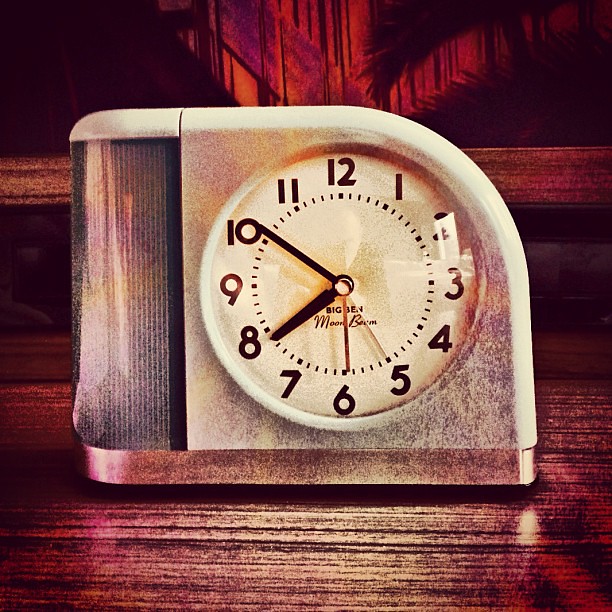This image features a vintage-looking clock, reminiscent of the 1960s, with a unique, asymmetrical shape. The clock has a primarily square form, but the upper right corner transitions into a circular design. The clock sits on a brownish wooden surface, likely a dresser, adding to its nostalgic charm. The clock face is circular and white, framed by a border that is white on the left while the bottom appears to have a bronze hue.

The clock displays black numerals and hands, including a minute hand, an hour hand, a second hand, and what seems to be an alarm arm. Below the hands, the text "Big Ben" and potentially "moonbeam" or "bigly" is partially visible. Despite the unclear text, the clock is set to 7:51:25, with the alarm seemingly positioned around 6 o'clock. Additionally, a feature on the right side could be a light, handle, or perhaps a speaker, though this is not easily discernible.

Enhancing its artistic feel, the image has a Photoshop effect that gives it a slightly painted appearance. Behind the clock, within the frame, there is a painting or decorative background piece with a red base and dripping black paint motif, contributing to the overall vintage aesthetic.